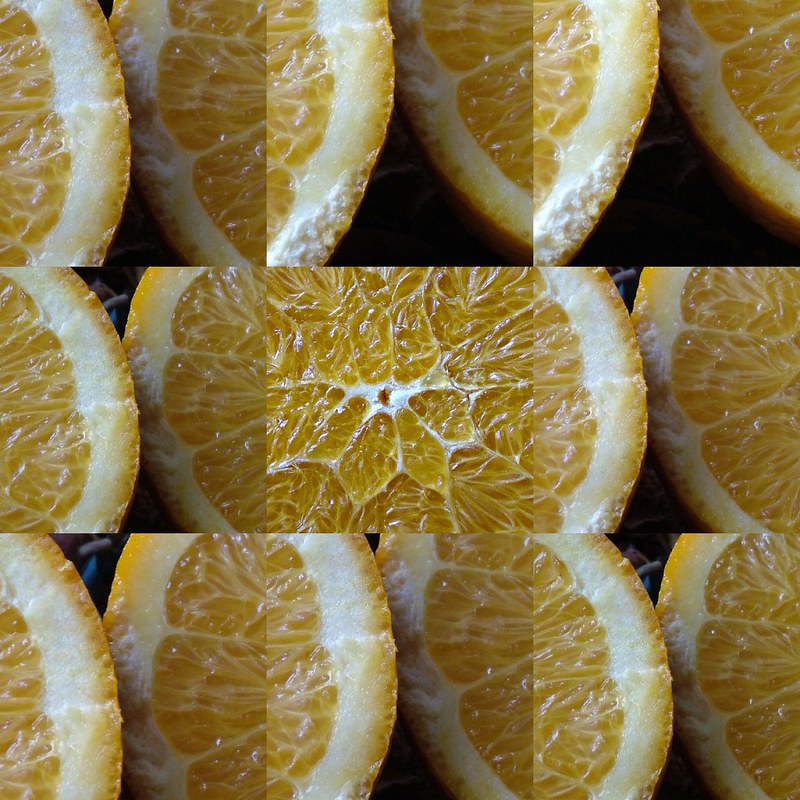This close-up photograph displays a lemon divided into a mosaic of nine square images arranged in a tic-tac-toe grid layout. Each square presents a different angle and lighting of the lemon, effectively fusing multiple perspectives into one cohesive image. The middle square showcases the lemon's inner pulp with a notable white central spot that resembles a spreading pattern. The surrounding squares feature varying degrees of brightness: the left column of images shows the lemon in darker shades, while the right column highlights it in a brighter yellow hue. This contrast accentuates the detailed textures of both the lemon's rind and inner flesh. The overall effect creates a jigsaw-like illusion, giving an intricate and multifaceted view of the lemon's surface and internal structure.